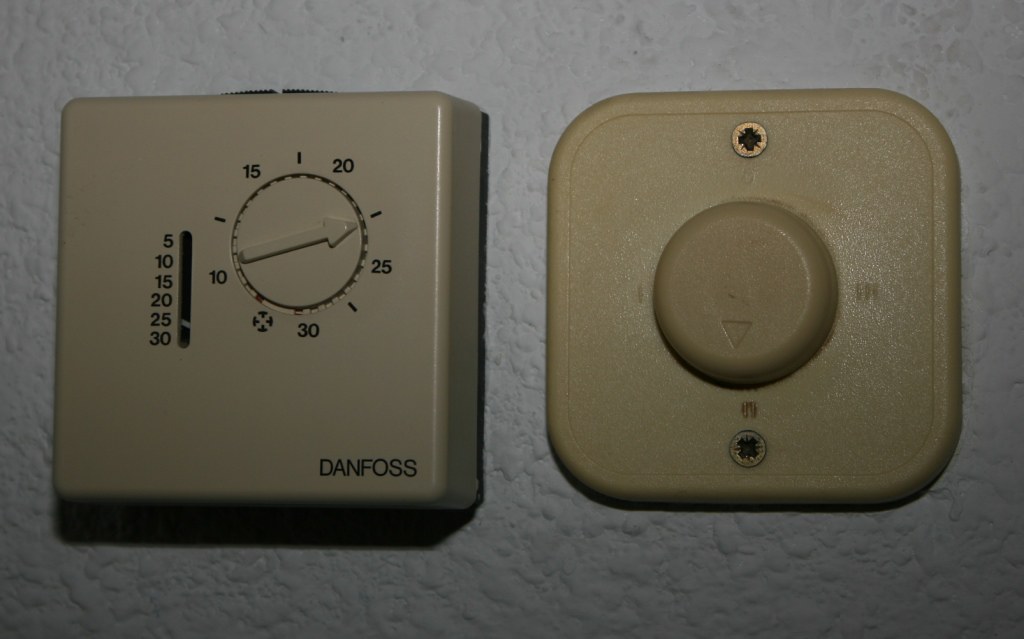The image depicts a dimly lit wall featuring two dials that appear to be part of a building's control system. The left dial resembles a thermostat, featuring a scale marked in black text ranging from 5 to 30, with the scale incrementing by 5 (5, 10, 15, 20, 25, 30). The dial has a cream white marker indicating its current setting, which lies between 20 and 25. The design includes a slider that appears as a gap, adding to its utilitarian aesthetic. On the right side, there is another similar object, although its dial lacks numerical indicators. Instead, it has an arrow pointing south. This second dial, also in a creamy, slightly brown shade, presents a minimalist appearance with no additional markings. The overall scene is quite dark, adding a sense of mystery and functionality to the setting.